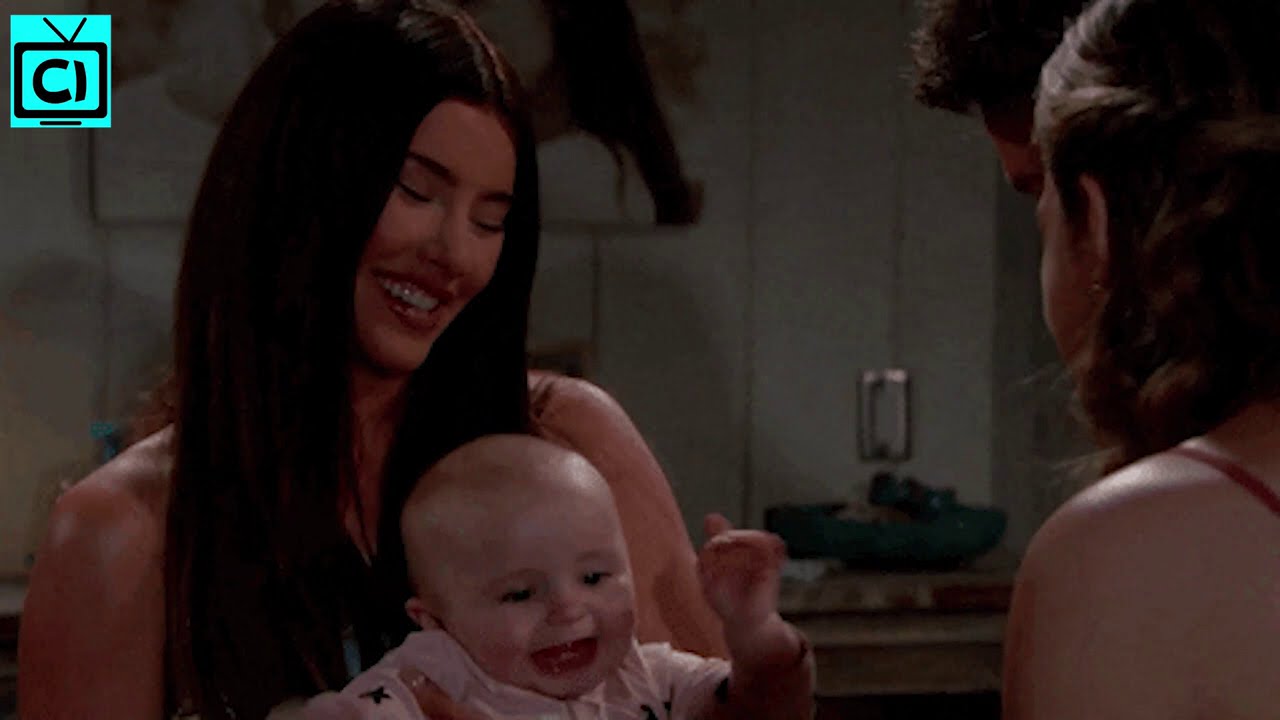The image captures a tender indoor scene involving four individuals. Central to the composition is a smiling woman with long dark hair, eyes either closed or gazing fondly downward as she holds a bald baby, who appears delighted with its arm raised. She is wearing a sleeveless shirt, revealing her shoulders and arms. Positioned in front of her is another woman, visible in profile with only her ear, side of her face, and shoulder discernible. She appears to be engaging with the baby as well. To the far right, partially obscured and identifiable by only the top of their hair, is another person, possibly male. The setting is a dimly lit room adorned with a painting and a bluish dish in the background. In the upper left corner, a closed-caption TV icon featuring a TV with an antenna and the letters 'CI' is faintly visible.